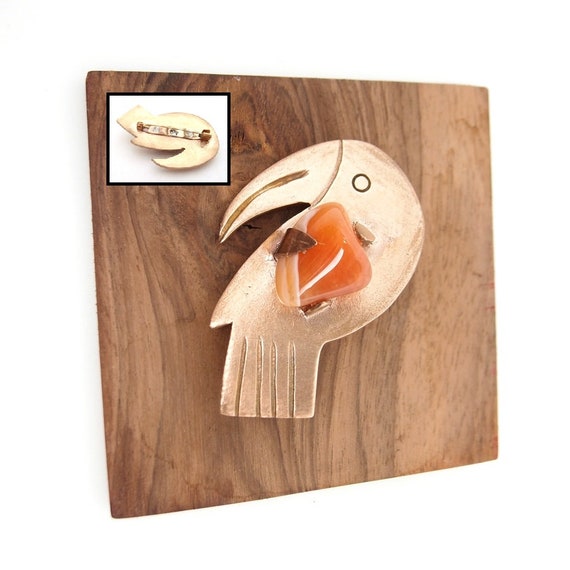The image depicts a gold bird pin lying on a wooden surface, plausibly a countertop or table, which extends vertically from top to bottom. The bird’s design features a broad body, long beak, and squared-off tail feathers. Notably, the bird has a black circular eye and an orange stone set in its center, secured by three clips. In the upper left corner of the image, there is a smaller section highlighting the back of the pin with its white background, revealing the pin's clasp mechanism. The color palette includes gold, brown, black, white, and orange tones. This artistic creation, possibly a vintage item, seems likely positioned for sale or display.